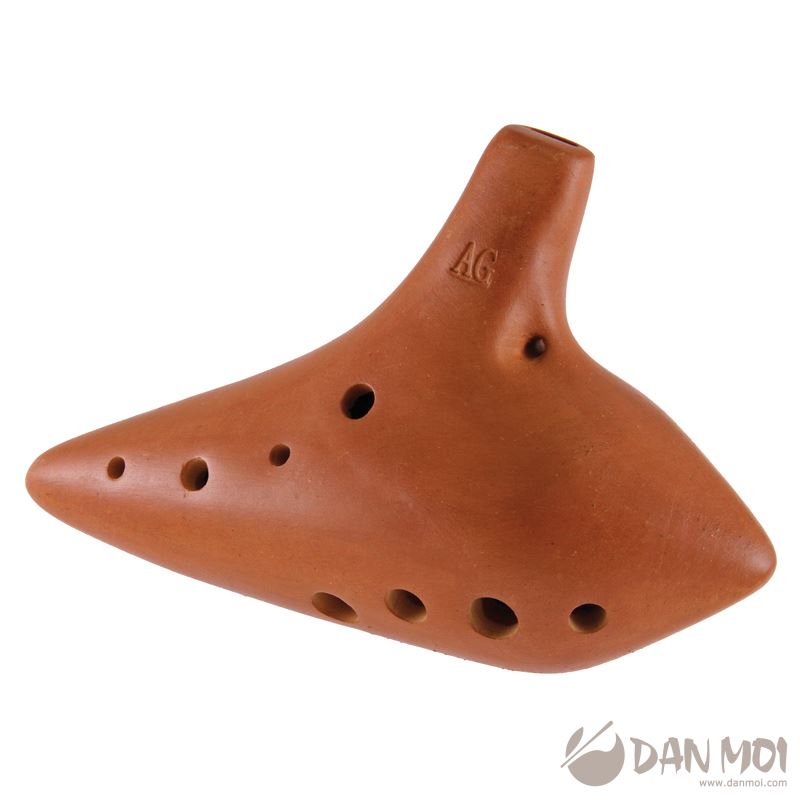The color photograph features an irregularly shaped object resembling the head of a golf club, carved out of wood with a distinct orangish hue. The object measures approximately three inches in length from left to right and has a football-like form with a one-inch stem extending from it. Engraved on the stem are the letters "A.G." The texture and tone of the object suggest it could be made of wood, although it has a terracotta-like color, varying from a lighter orange on the front and back to a darker orange on the side facing the viewer. 

The object’s triangular form points towards the left, with several holes of alternating sizes running across the toe portion, from small to slightly larger. Additionally, there is a single hole on the back of the heel and four more on the bottom side, providing a unique pattern of perforations. The photograph is set against a white background, enhancing the detailed texture and color variations of the object. At the bottom right corner, there is a small gray logo that reads "Dan Moe," accompanied by an illegible URL. The image captures the object with photographic representational realism, emphasizing its intricate design and vibrant color.